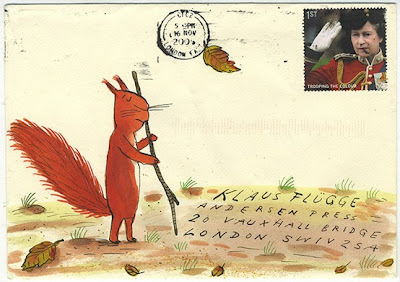The image shows a small, horizontally-aligned, rectangular envelope or postcard, which appears aged with a yellowed and weathered look. In the top center, there is a faint black postmark that is difficult to read. Adjacent to this is a stamp in the upper right corner, featuring a prince-like figure or a person in a military or marching band uniform, dressed in red and gold with white gloves and a black hat. Overlaying the envelope is a whimsical illustration. On the left, a squirrel, standing on its hind legs with eyes closed and holding a stick, has presumably written out the address. The addressee is Klaus Flugge, F-L-U-G-G-E, Andersen Press, 20 Vauxhall Bridge, London, SW1V 25A. The ground in the illustration is adorned with fallen leaves and grass, and a yellow-brown leaf is positioned overlapping the black postmark at the top center.